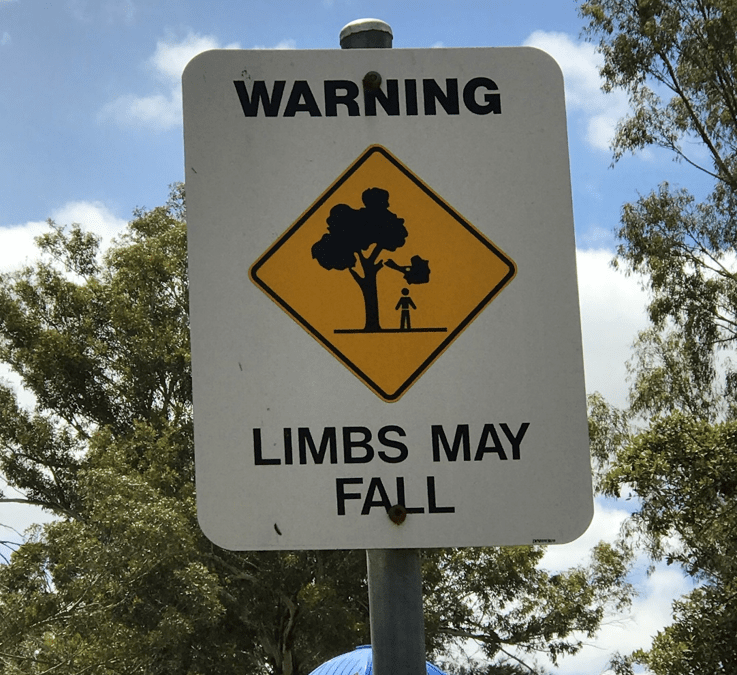The image depicts a brightly lit outdoor scene with a clear blue sky and scattered white clouds, framed by tall green trees on both sides. At the center stands a vertically aligned rectangular warning sign affixed to a silver or gray metal pole with rusted screws. The sign has a white background and features the word "WARNING" in bold, all-caps black letters at the top. Below this, there is a diamond-shaped yellow icon outlined in black, showing a tree with a falling branch about to strike a person standing beneath it. Further down, the sign cautions "LIMBS MAY FALL" in uppercase black letters. The overall clarity and brightness of the image emphasize the details and the atmospheric daytime setting.